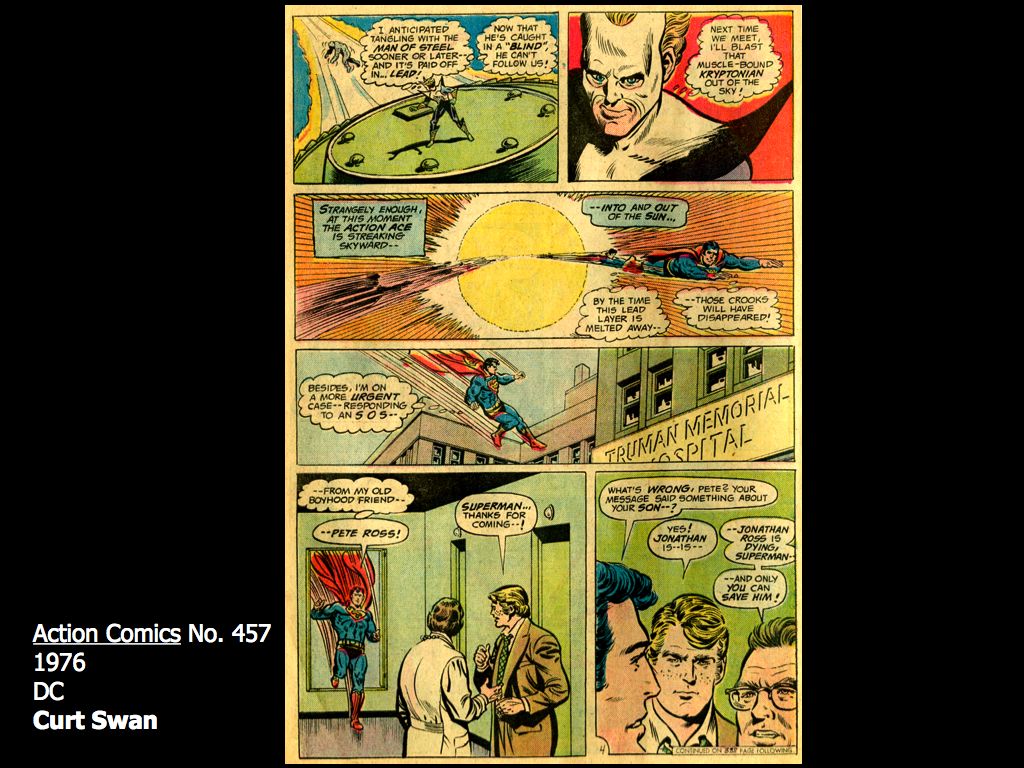The image is a large, solid black square with a comic strip perfectly positioned in its center. In the bottom-left corner, white left-aligned text indicates "Action Comics," underlined, followed by "number 457," "1976," "DC," and "Kurt Swan" in bold. The comic strip itself is composed of six panels in a combination of rectangular and square shapes. At the top, a villain against a green background boasts, “I anticipated tangling with the Man of Steel sooner or later, and it's paid off in lead, now that he's caught in a blind, he can't follow us.” Adjacent to this, a close-up of the villain declares, “Next time we meet I'll blast that muscle-bound Kryptonian out of the sky.” In the middle section, a large rectangle shows Superman flying. Below it, another rectangle depicts Superman landing at "Truman Memorial Hospital." In the bottom sections, Superman crashes through a window and exclaims, "Pete Ross!" Pete, in a suit, responds, “Superman, thanks for coming.” In the final panel on the lower right, Superman asks, “What’s wrong, Pete? Your message said something about your son,” to which Pete replies, “Yes, Jonathan Ross is dying, Superman, and only you can save him.” The comic's vibrant colors include shades of black, white, yellow, blue, red, purple, orange, and green.